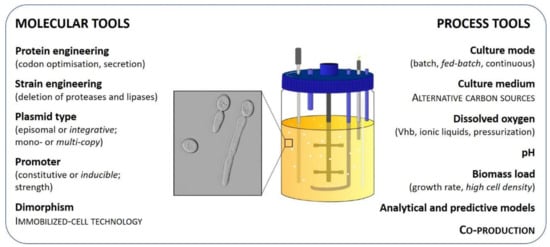This scientific diagram with a white background and grey rounded rectangle outline features a central canister filled with a yellowish liquid up to two-thirds of its height. The canister has a blue top with various tubes protruding into the liquid. Within the liquid, a small highlighted square is zoomed out to a grey square showcasing microbes or small particles.

On the left side, a column titled "Molecular Tools" lists headings: protein engineering, strain engineering, plasmid type, promoter, and dimorphism. On the right side, a column titled "Process Tools" includes headings: culture mode, culture medium, dissolved oxygen, pH, biomass load, analytical and predictive models, and co-production.

The diagram effectively illustrates the interaction between molecular and process tools in a biotechnological or microbiological setup.